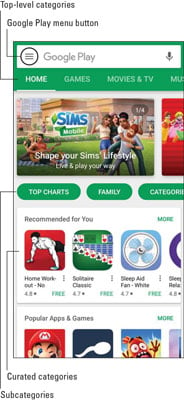The image is a detailed layout of the Google Play interface. In the upper left corner, there is a section labeled "Top-Level Categories," with a line extending downwards and slightly to the right, connecting to the word "Home." Immediately below "Top-Level Categories," the phrase "Google Play Menu Button" is displayed, with another line descending from the letter "G" towards the right, ending at a circle. 

Positioned beside this is an open search bar containing the text "Google Play." Continuing from the word "Home," which is underlined, the categories "Games," "Movies," and "TV" are listed. The image highlights the game *The Sims Mobile*, showcasing its characters in a vibrant, grassy area. Two Sims are depicted sitting on a picnic blanket, with one holding a guitar. A large building and some bushes provide a scenic background. The caption reads: "The Sims Mobile. Shape your Sims lifestyle. Live and play your way."

Below this section, a label "Top Charts" appears, with a line stretching from it towards the left, running down to the bottom of the screen, leading to "Subcategories." Further down, another label, "Recommended for You," is displayed next to an image of a man performing a push-up, marked by a red square. A line extends leftward from this image, continuing to the bottom where it says "Curated Categories." 

At the base of the screen, the "Popular Games and Apps" section is shown, featuring an image of Super Mario winking, with his iconic red hat.